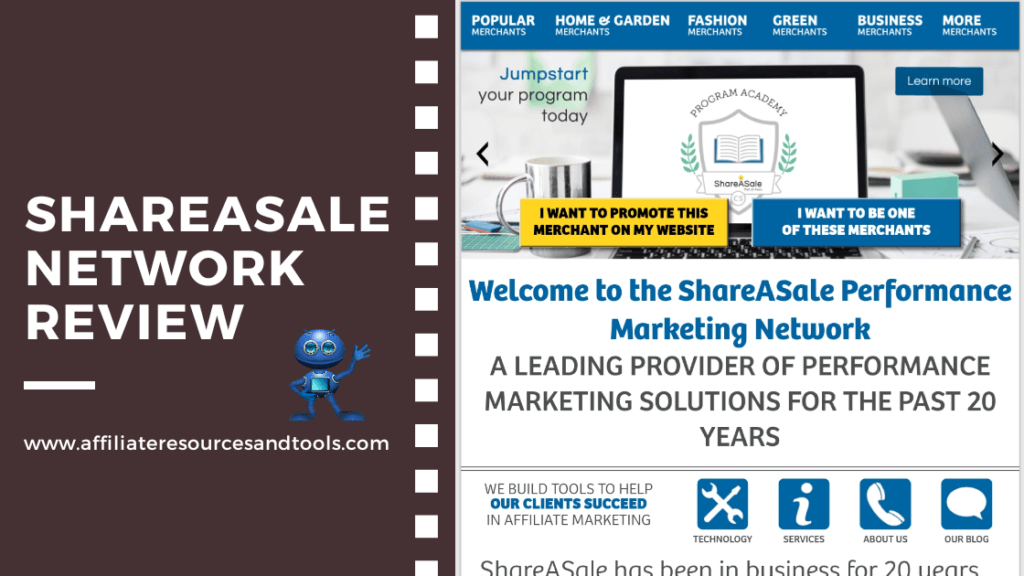The image features a predominantly brownish-purple rectangle on the left-hand side, which includes various elements that contribute to its detailed layout. Starting from the top, it prominently displays the text "Share a SAIL Network Review" followed by a horizontal white line. Below this, there's an illustration of a small blue man, accompanied by a website link. The background is accentuated with an array of white squares arranged to resemble a strip of film, enhancing its visual appeal.

Transitioning to the right-hand side, a blue rectangle contains several labeled tabs: "Popular," "Home and Garden," "Fashion," "Green," "Business," and "More." Despite the smaller font rendering some of the text illegible, the sections indicate a well-organized structure. Further down, the blue text "Jump Start" draws attention, followed by the phrase "Engage Your Program Today" beneath it. Adjacent to these, there are images depicting a coffee cup, a desktop computer with the words "Program Academy" and an associated emblem.

Further down the image, another blue rectangle on the right implores viewers to "Learn More," paired with a hard-to-discern picture. Below this, a vibrant yellow rectangle with bold black text reads "I want to promote this merchant on my website." Subsequently, a blue rectangle states, "I want to be one of these merchants" in white text, followed by a welcoming message in blue: "Welcome to Share a SAIL Performance Market Network." In black text just below, it highlights the company's longstanding expertise: "A leading provider of performance market solutions for the past 20 years."

A striking black line partitions this section, succeeded by another separator featuring a gray gradient. It further emphasizes the company's mission: "We build the tools to help our clients succeed in affiliate marketing." Within this segment, images of various tools are included, though finer details remain indistinguishable. The design features a cursive "I" in another blue square with white illustrations, continuing the consistent aesthetic. Additional blue squares house icons of a telephone and a speech bubble, while some accompanying text is truncated at the bottom of the image, leaving the full message incomplete.